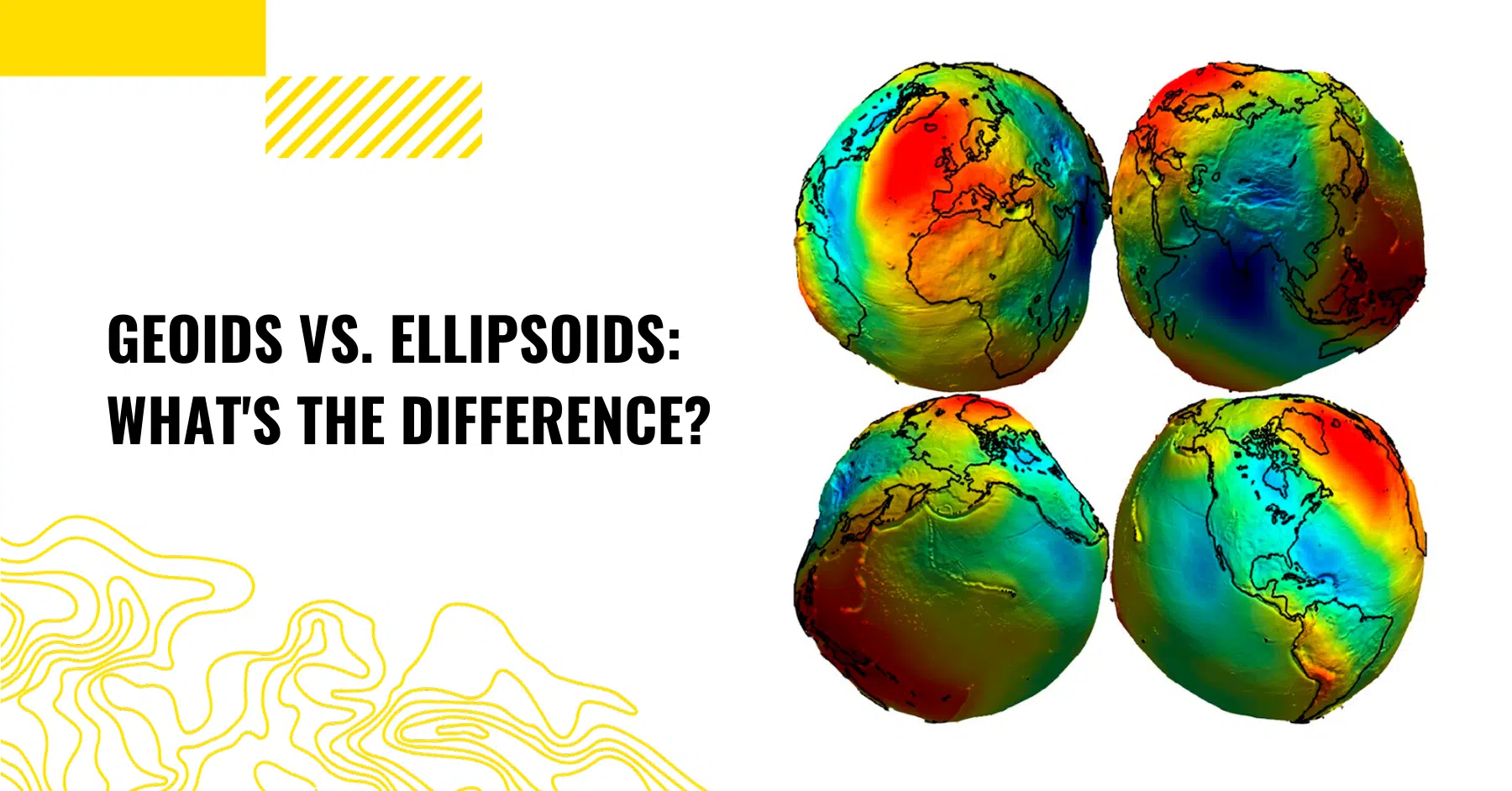The image is a detailed diagram comparing geodes and ellipsoids. It features a white background with a yellow design on the top left, consisting of rectangles and squiggly lines, and a similar design on the bottom left. In the middle left, bold black uppercase text reads "GEODES VERSUS ELLIPSOIDS: What's the difference?" To the right, the diagram displays four misshapen, rainbow-colored representations of Earth, highlighting variances in temperature. Each Earth-like sphere is adorned with heat maps in shades of red, orange, yellow, green, and blue, showing different temperature zones. Distinct continents can be seen, including Africa in the top left, Asia in the top right, North America at the bottom, and a portion of the Southern Hemisphere to the left.